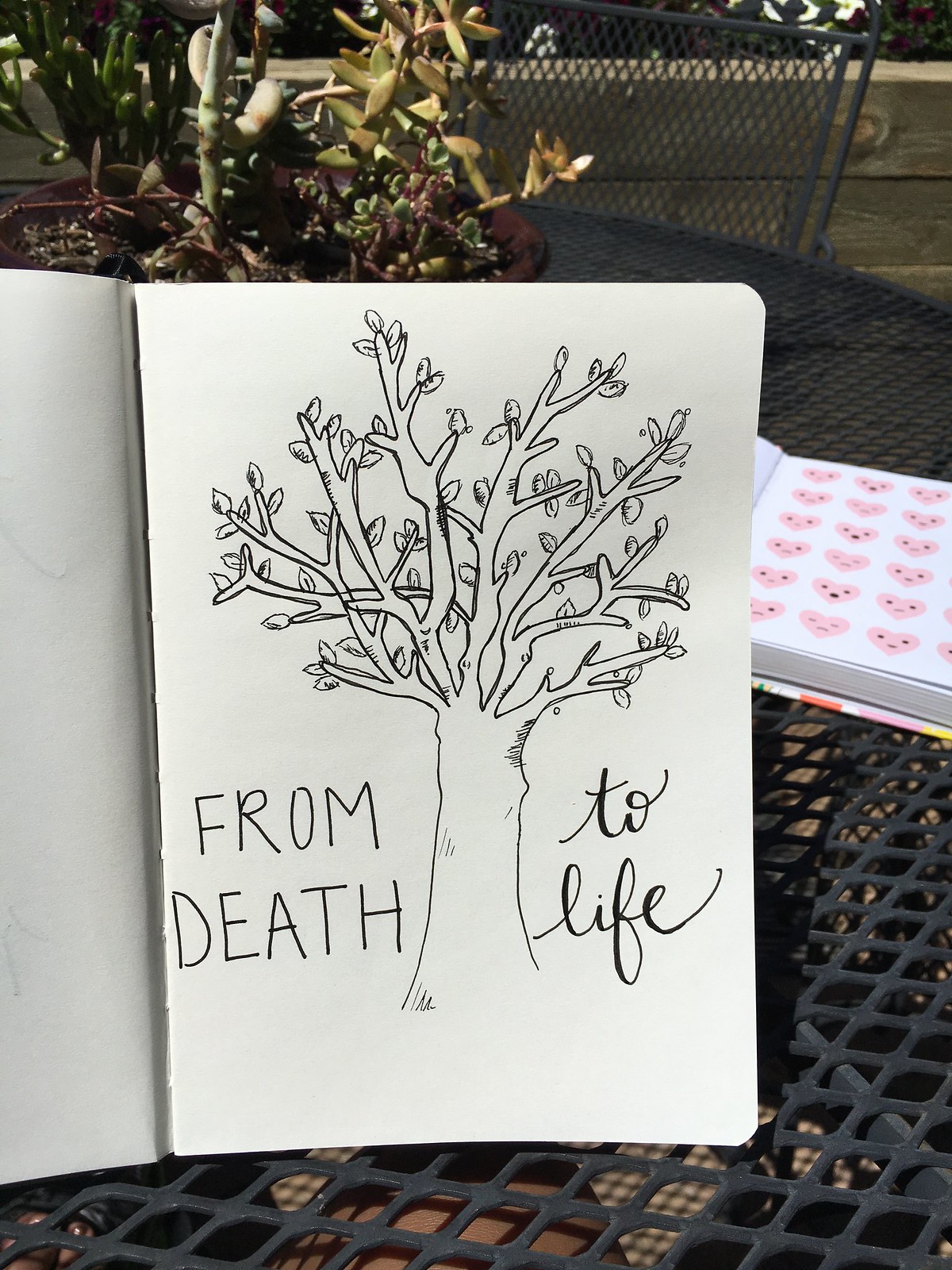A detailed black pen drawing rests on a white piece of paper inside an open sketchbook, which is propped up on a metal grate patio table outdoors. The drawing depicts a tree with numerous branches, each adorned with fresh leaves. On the left side of the tree, the phrase "FROM DEATH" is printed in bold capital letters, while on the right side, the phrase "to life" is written in delicate lowercase cursive. In the background, another open book is visible, featuring heart stickers with various facial expressions. Beside the sketchbook, a potted plant can be seen on the table, adding a touch of greenery to the serene outdoor setting.